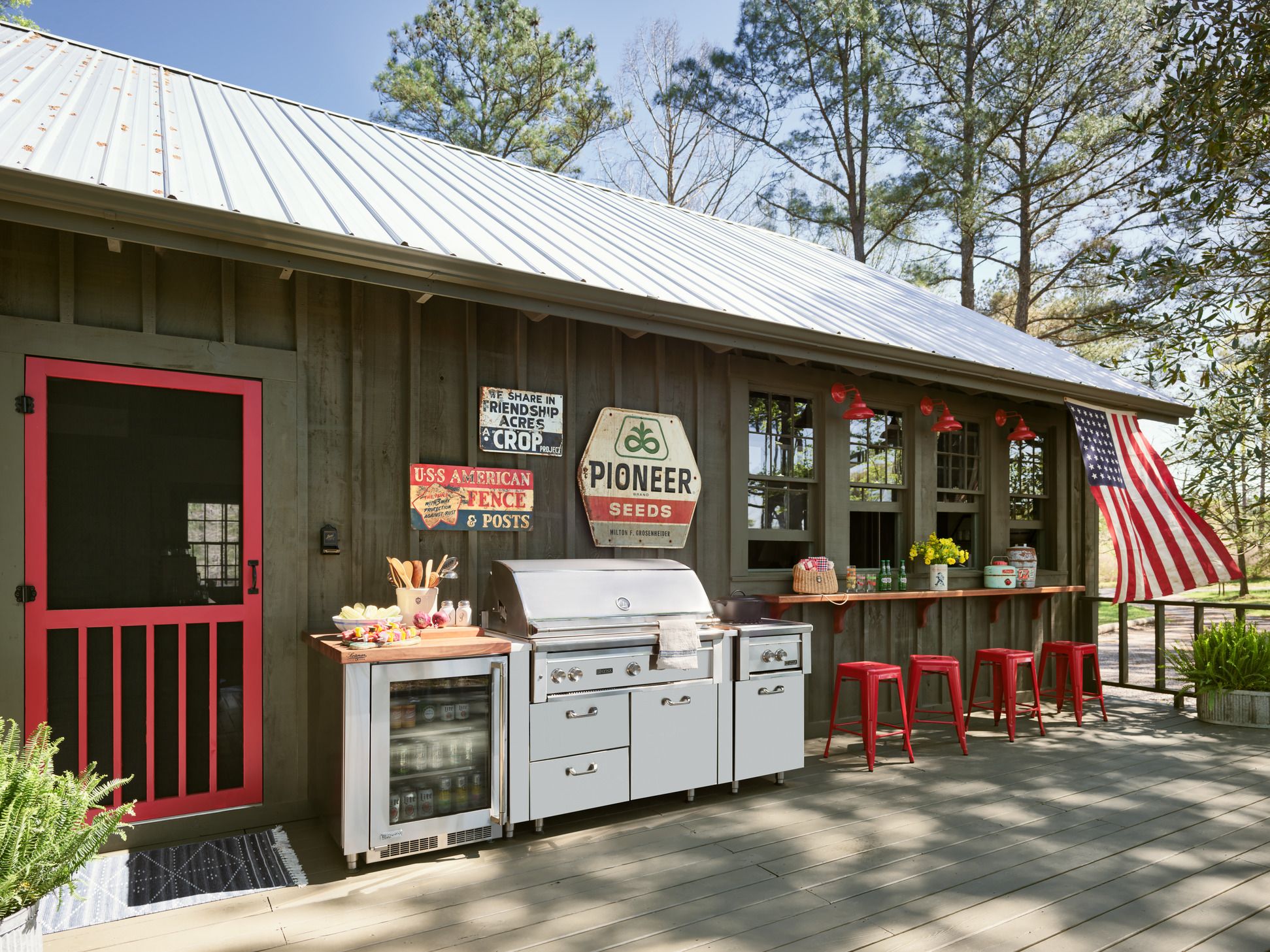The image depicts the exterior of a quaint, single-story wooden diner, reminiscent of a chalet, nestled in a wooded park area. The building, painted a dark green, is accented with red features including a frame fly screen door, cafeteria-style stools, and various decorations. The diner has a charming old-fashioned yet modern appeal, emphasized by vintage metallic signs that read "Pioneer Seeds," "Sharing Friendship Acres," and "USS American Fence and Post," which are mounted above a stainless steel outdoor barbecue. This well-equipped barbecue area, featuring barbecue tools, food, and a refrigerator stocked with canned drinks, is situated next to the red stools, which face a serving bench positioned in front of windows open to the outside. An American flag proudly hangs from the metal roof, adding to the inviting atmosphere. The setting is enhanced by the presence of decking in front of the building and a backdrop of lush trees, reinforcing the rural and serene ambiance.